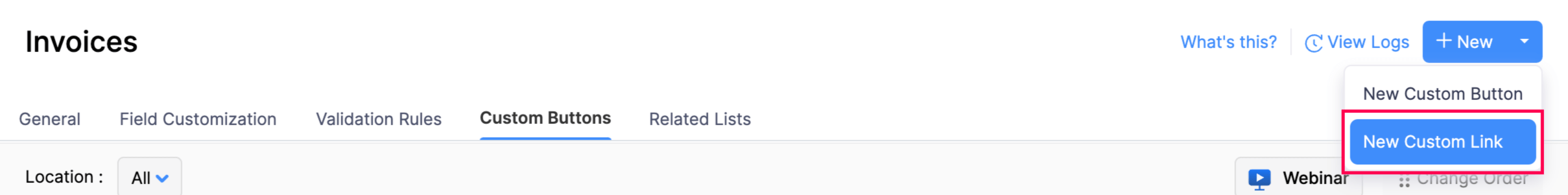This image displays a computer screen featuring an invoices interface. The screen has a white background with various text elements. In the upper left corner, the word "Invoices" is prominently displayed in black. Moving to the right, a blue text reading "What’s This?" accompanied by a question mark appears. Beside it, there is another blue text labeled "View Logs," followed by a blue button labeled "+ New" with a drop-down arrow.

This drop-down menu has been expanded to reveal two options: "New Custom Button" and "New Custom Link," both in blue text. The "New Custom Link" option is highlighted with a red rectangle. Beneath these options, on the left side, there are headings for different sections: "General," "Field Customization," "Validation Rules," "Custom Buttons," and "Related Lists," with the "Custom Buttons" section underlined in blue.

Further down on the left side, the word "Location" appears with the option "All" accompanied by a drop-down arrow. To the right side of the screen, there is an icon resembling a computer monitor. Adjacent to the monitor icon, the word "Webinar" is visible. Additionally, there seems to be a partial text mentioning "change," but the rest of the phrase is obscured by the drop-down menu at the top.